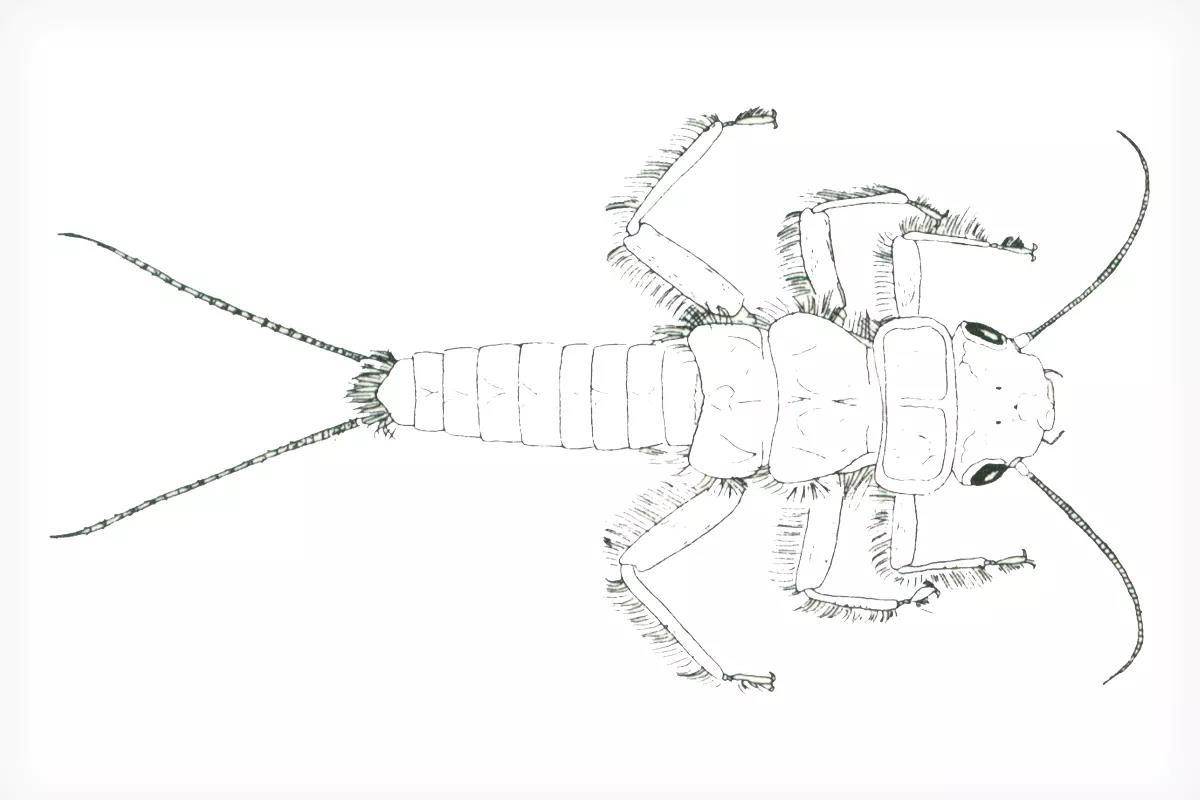The image is a detailed black and white drawing of an insect, rendered in pen and ink or pencil. It appears to show a nymph stage of an insect, exhibiting features resembling a cross between various species, such as a grasshopper, a scorpion, and a cockroach. The illustration is a top-down view, with the insect facing to the right, resulting in its head on the right side of the page and its tail on the left.

The insect's elongated body is segmented, boasting around eight to ten sections. At the rear, the tail culminates in two long, strand-like structures that resemble antennae but are part of the tail, anchored at a frilled base. The body also has six jointed legs, each adorned with small hairs, with hind legs longer than the front pairs.

The head of the insect has large eyes and curved antennae that sweep back from under the eyes. There are small mandibles extending from the mouth. The high-quality sketch captures intricate details, including the texture of the scales on the elongated tail and the hairs at the tail's end. The background is white, devoid of any text or additional objects, emphasizing the insect itself, making the drawing resemble a study in a scientific journal or a detailed book illustration.